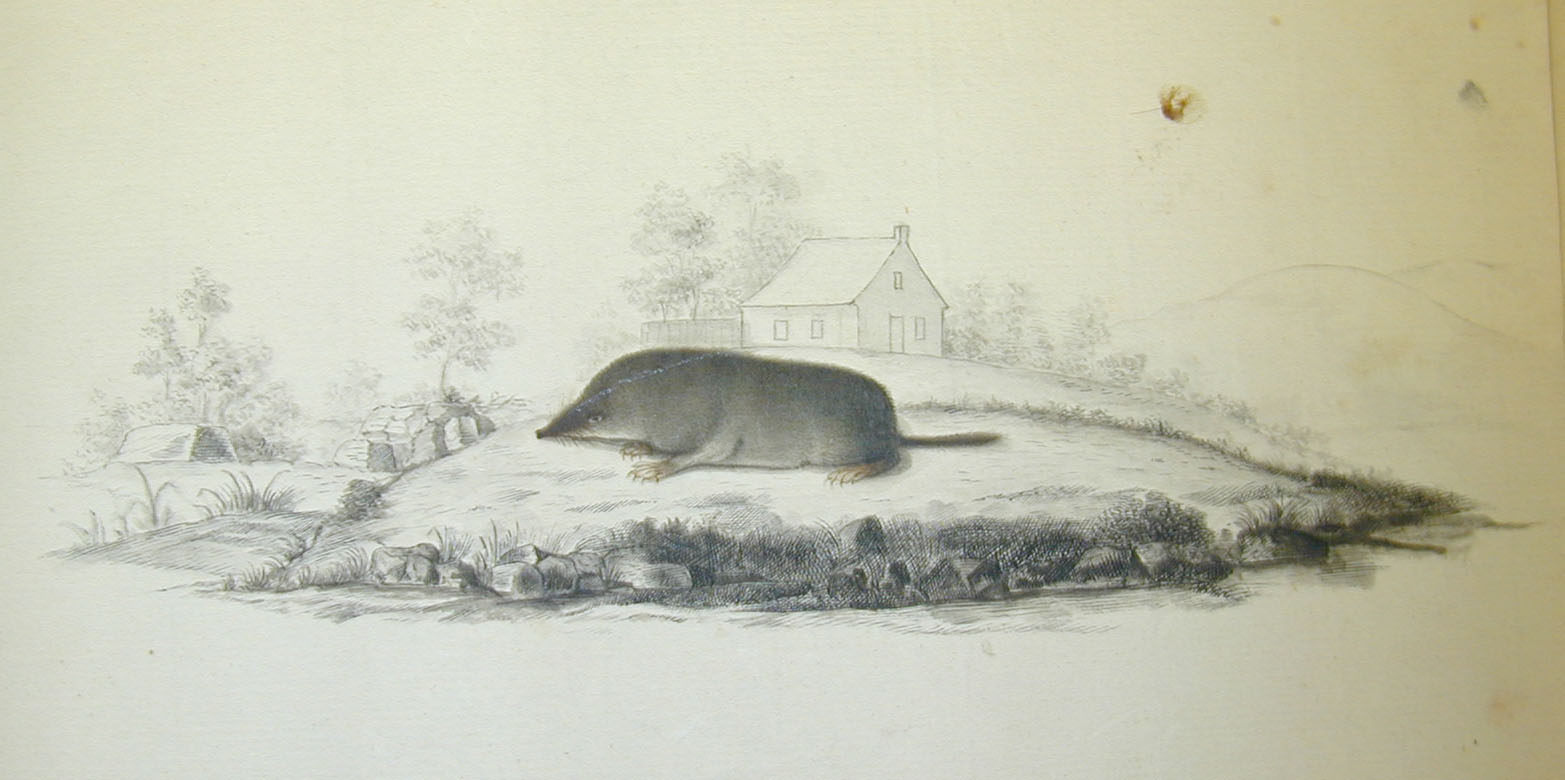This detailed black and white drawing depicts a sizable, furry rodent-like creature lying on the ground in the center of a small island, looking towards the left. The animal, resembling a large rat or possum, has a prominent snout, claws, whiskers, a tail, and is shaded in grey with some brown on its claws. Surrounding the creature is a well-detailed environment consisting of a house with four windows, a door, and a chimney situated on top of a hill. To the left of the house, there's a small barn or structure, also sketched. The island features rocks at the creature's base, grassy areas, scattered trees, and hills—larger ones on the right side—while water surrounds the entire scene, enclosing this intricate island setting. The imposing rodent-like creature, possibly the focal point of this artwork, captures attention with its unusual size and presence.